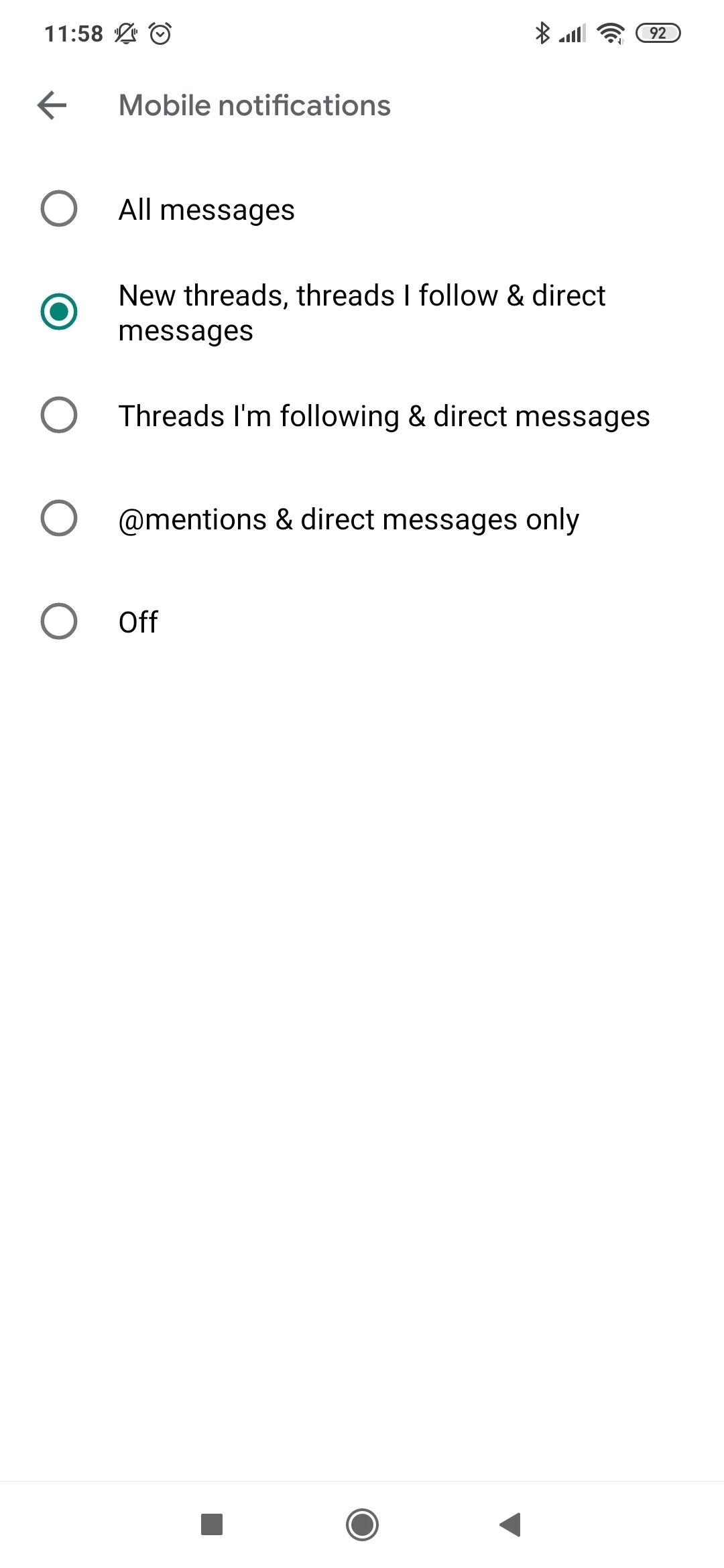The image displays a smartphone screen with various indicators and settings. At the top of the screen, the time is shown as 11:58. The ringer is muted, as indicated by the ringer-off icon. The screen also shows the clock and alarm settings. On the right side, icons indicate that the device is connected to Bluetooth and Wi-Fi, with the Wi-Fi signal strength being strong. Next to the Wi-Fi icon, the battery level is displayed at 92%.

Below these icons, the screen shows mobile notifications settings. A back arrow is visible at the top. The settings include the following options: "All messages," "New threads, and threads I follow in direct messages," "Threads I'm following and direct messages," "@mentions and direct messages only," and "Off." 

Currently, the "New threads and threads I follow in direct messages" option is activated. Each of these notification options is evenly spaced, although the spacing above the "All messages" option is slightly wider than the others.